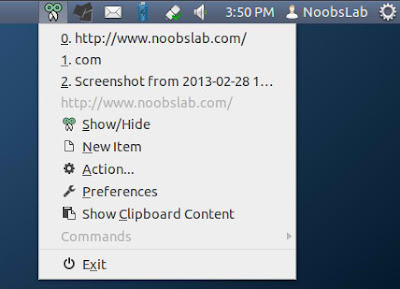This image displays a detailed interface of an application, likely a screenshot tool or a utility dashboard. The top of the interface features a row of icons starting with a pair of scissors icon with green handles, suggesting a cutting or screenshot function. Right next to it, there are various icons including multiple squares scattered randomly, an envelope, a blue bottle, a book, and a speaker, indicating different functionalities or apps. 

At the top-right corner, the current time is displayed as 3:50 PM, and beside it, there's a cartoon character that might represent a user profile or avatar. Below these elements, the application prominently displays a link "http://www.nubslab.com/1/2/screenshot2013-02-28" indicating it might be tied to a web service or an archived screenshot from the aforementioned date.

Further down, there are options labeled "Show/Hide” alongside the scissors icon. Another row includes icons such as a page with a label "New Item,” a settings gear labeled "Action," a flyers icon labeled "Preference," and a clipboard with a page that states "Show Clipboard Content." 

At the bottom of the interface, there's an "Exit" option, hinting at its role for closing the application or dashboard. The branding "Nub's Lab" or "Nubs Slab" is mentioned within the application, tying the functionalities to this specific developer or service.